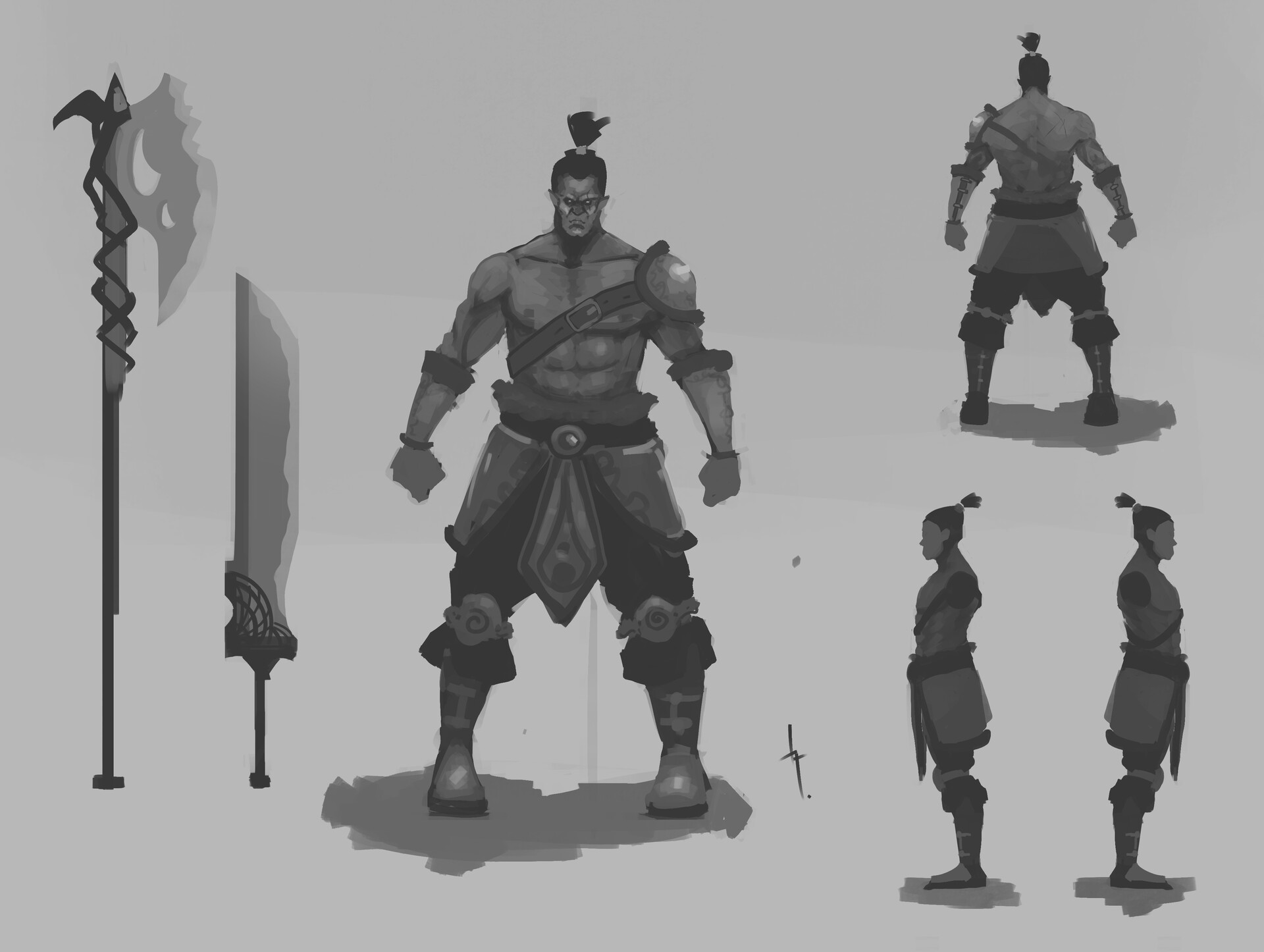This horizontal, rectangular image, rendered in black, white, and shades of gray, resembles a detailed drawing or possibly a computer-generated artwork. Dominating the center is a muscular, shirtless warrior with a leather strap across his chest and various pieces of armor-like clothing, including tall boots. His distinctive hairstyle features hair sticking straight up. To the left of him, you see two weapons: a long axe and a large sword. In the top-right corner, the warrior is depicted from the back, while in the bottom-right corner, he is shown in both left and right profile views. These additional renderings suggest a preparatory sketch for a cartoon or animation, giving multiple perspectives of the same character. There is no text present in the image, and the entire composition uses a monochromatic color scheme, enhancing its stark and dramatic appearance.